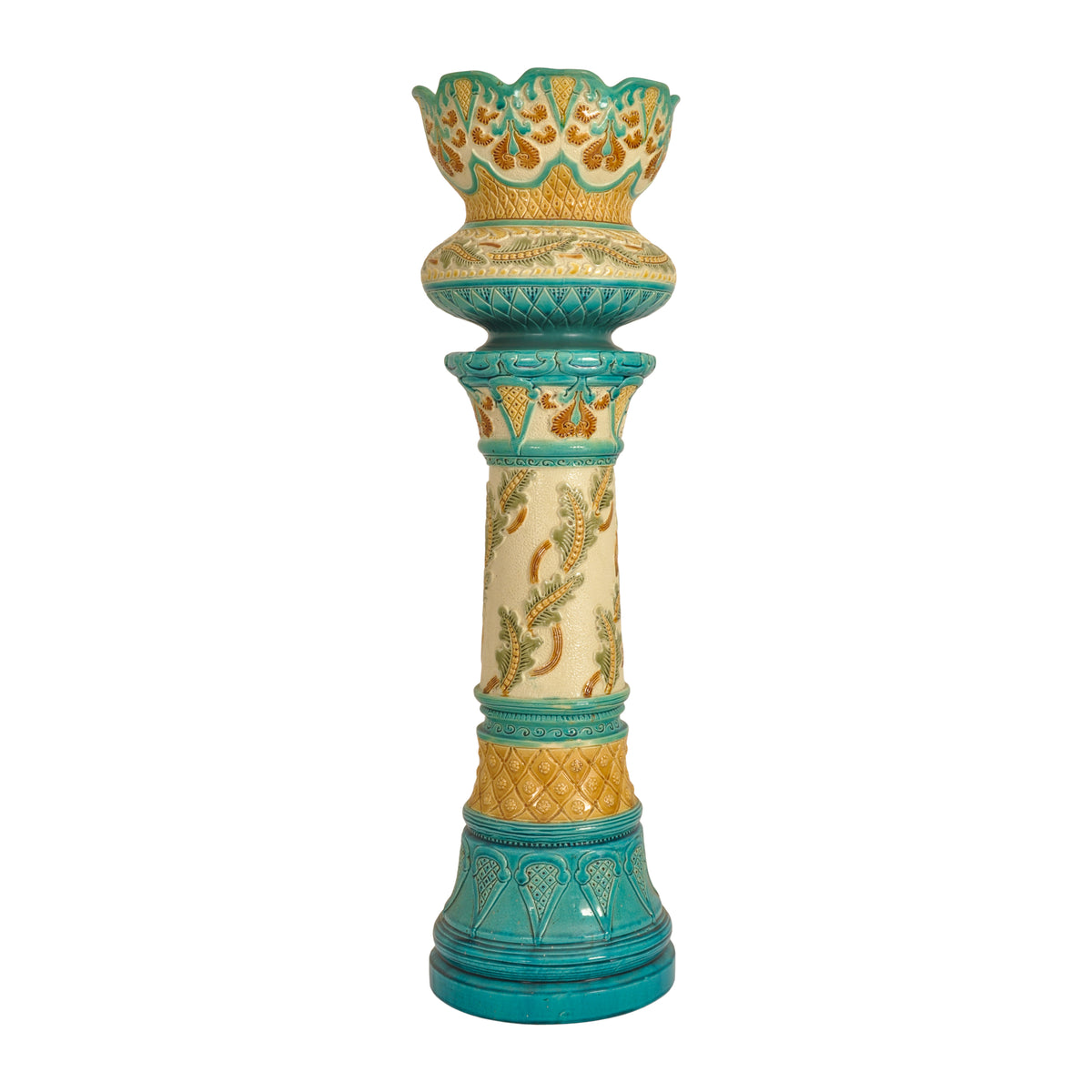This image showcases a detailed and colorful vase that appears to be crafted from fired clay. The vase is predominantly adorned with hues of blue, light blue, golden yellow, beige, olive green, and light brown. Its design starts with a top section that flares out into a unique, scalloped rim resembling a lotus flower, adorned with intricate engravings that include floral motifs, plant-like emblems, and honeycomb patterns.

As the eye moves down the vase, its long, slender body is decorated with a central design reminiscent of floating bacteria or parasites with a beige body and green accents. This part of the vase features a bulb-like shape that recalls the top of a staircase handrail or the contours of a chess piece, specifically a pawn.

Further down, the base of the vase broadens out with swirls and vibrant colors, predominantly in shades of yellow and orange, giving it the appearance of a stable, supporting structure. The overall design suggests both a functional and decorative art piece, resting against a stark white background that emphasizes its vivid and intricate detailing.